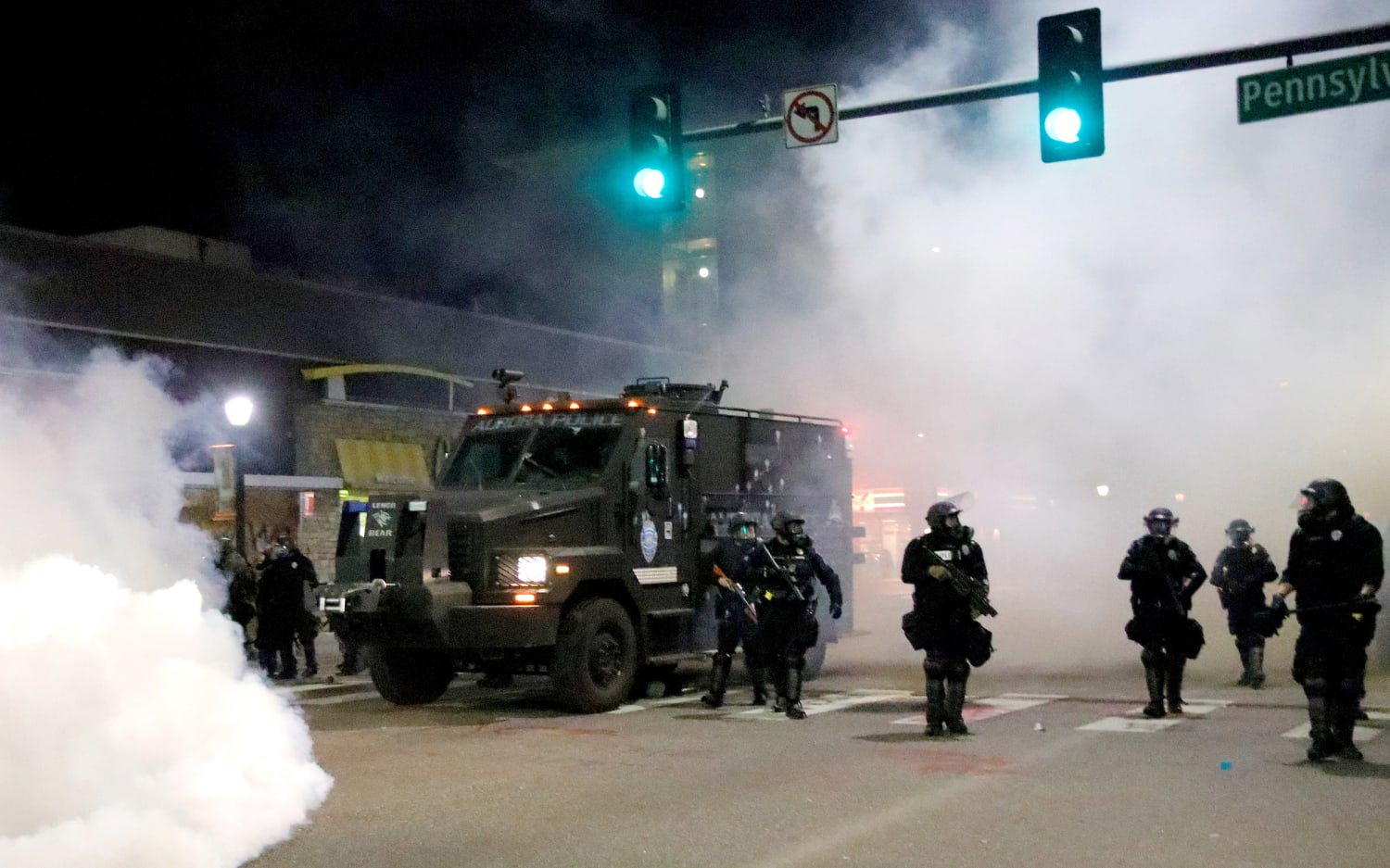The image depicts a chaotic nighttime scene where approximately half a dozen uniformed police officers in heavy tactical gear and helmets are responding to an event, possibly a riot. They are equipped with military-grade rifles and dressed in black, standing around a heavily-armored SWAT vehicle marked "Aurora Police." The officers and the vehicle are positioned under two green traffic lights at an intersection marked by a partially visible street sign reading "Pennsylvania," suggesting the location might be Washington, D.C. There is a "No Left Turn" sign hanging between the traffic lights. The immediate area is enveloped in thick clouds of smoke or tear gas, obscuring much of the surroundings, including a nearby McDonald's illuminated in the background. The scene is further shrouded in fog to the left and right, intensifying the atmosphere of confusion and tension. The officers are standing on a gray street with visible white crosswalk lines.